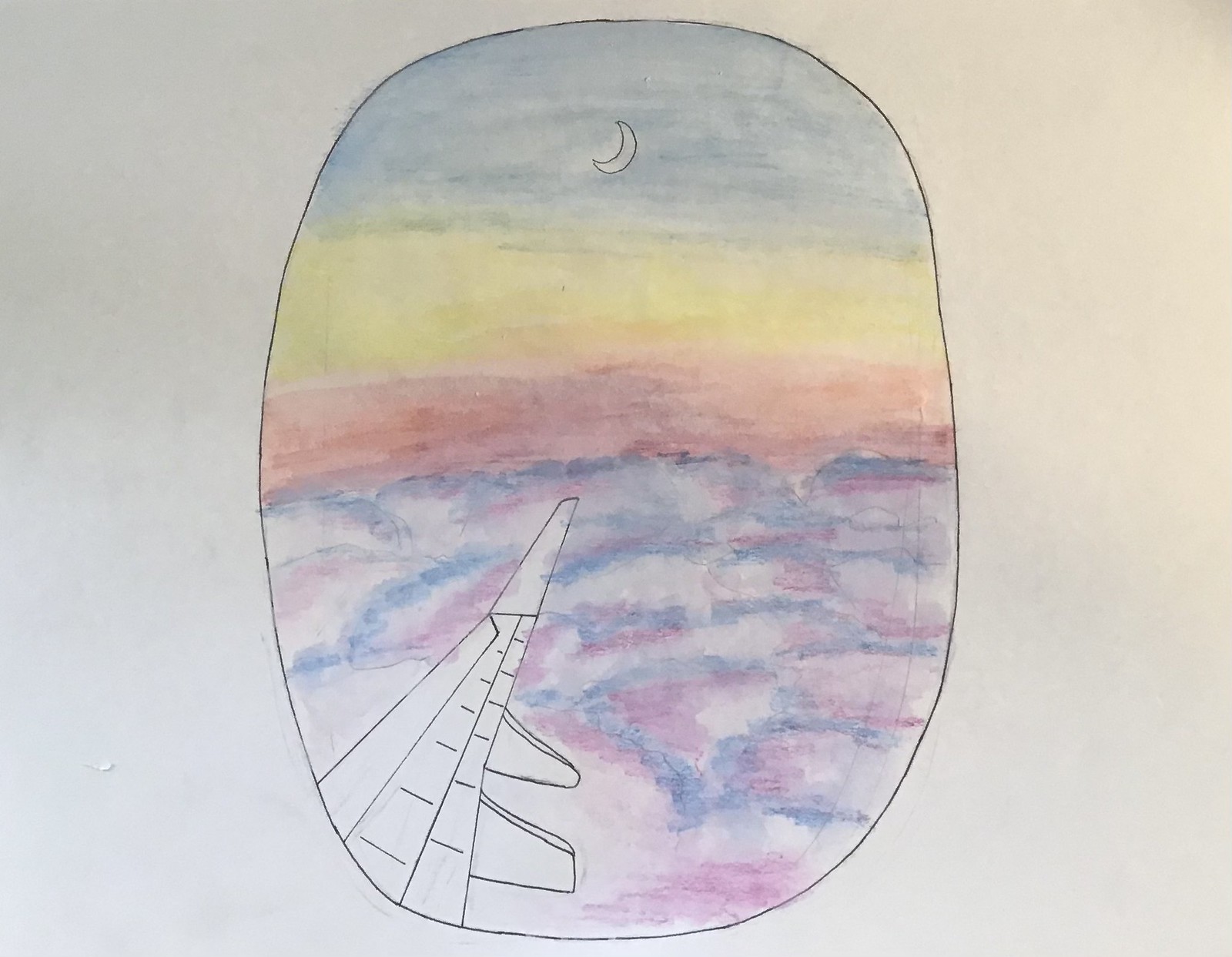This image captures a captivating watercolor painting solely on the plain white background of the paper, devoid of any table or wall context. At the center of the composition, a sizable oblong shape representing an airplane window dominates the scene, occupying about three-fourths of the page. Inside this window, the viewer is treated to a serene sunset landscape. The sky is beautifully rendered in bands of color, transitioning from a deep blue at the top, which houses a delicate crescent moon, fading through shades of yellow and culminating in a warm orange halfway down. Below this gradient sky, fluffy clouds of dark blue-purple and magenta float serenely. In the bottom left quadrant of this window, a meticulously detailed portion of the airplane's wing stretches into view, sketched in precise pencil or pen lines without any added color. The composition effectively captures the ethereal beauty of a sunset seen from an airplane, highlighting the soft, flowing washes of watercolor and the sharp contrast of the monochromatic wing.